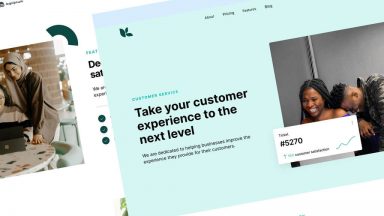In the top left corner of the image, a small, indistinct logo is visible. The background of the image is predominantly white. Beneath this logo, there is a photograph featuring a woman wearing a taupe-colored hijab. The woman has on a long-sleeved, baggy brown shirt and appears to be leaning on a basic white tabletop with a possibly painted floral print. She seems to be leaning towards her right, possibly embracing another person next to her. In the background, a brick wall and a railing are visible, and the woman might be wearing white pants.

Towards the upper right of the image, a thick, dark teal semi-circle frames the corner. Next to this, in blue writing, there appears to be the word "SEAT," although it is not entirely clear. Below this, in bold black text, the letters "DE" are visible, followed by the word "SAT." Below these bold letters, there are two lines of smaller black text, and beneath these lines are three large, bold bullet points that match the teal color of the framing curve.

Superimposed on this image is a screenshot of a webpage. The top header of the webpage is light blue, while the rest of the page has a very light aquamarine background. In the upper left corner of the webpage is a logo comprised of three different teal leaves. The left leaf is large, the middle leaf is small, and the right leaf, slightly larger than the middle one, completes the trio.